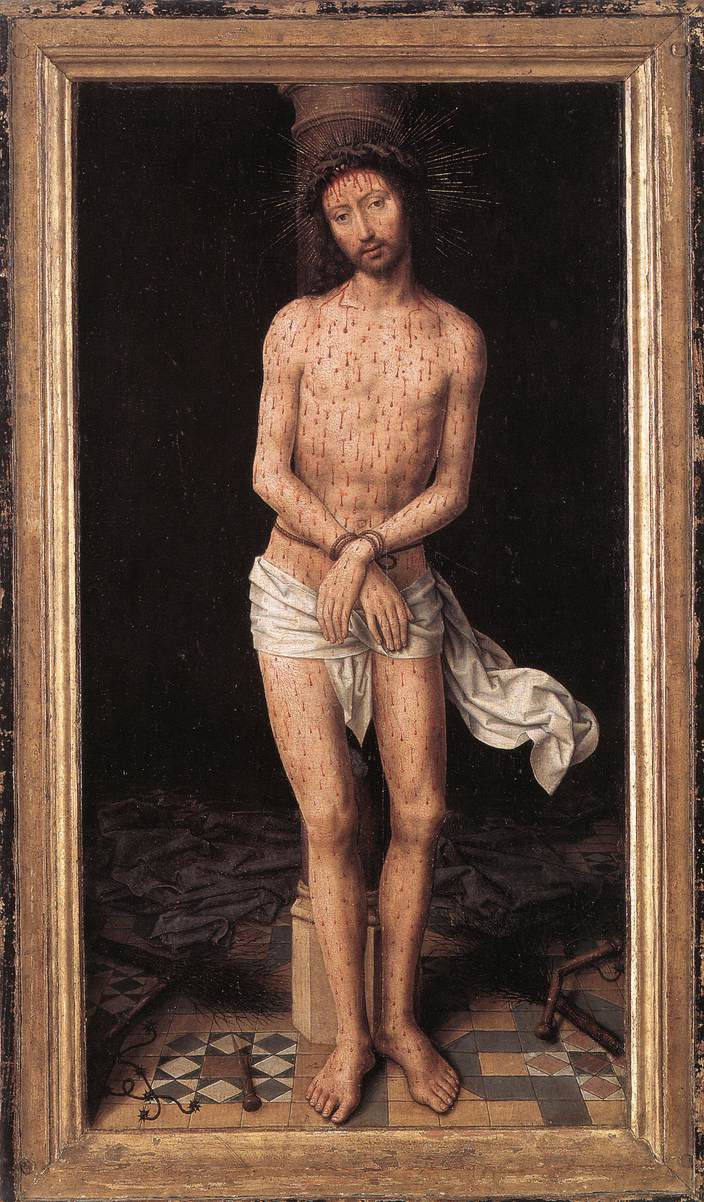This vertical rectangular painting, encased in a brown wooden frame, portrays a thin, white man who appears to be a depiction of Jesus Christ. The background of the painting is very dark, almost completely black, which starkly contrasts with the figure in the center. The man is standing barefoot on a tile floor with hues of orange, brown, and gray. He is nearly naked, with only a white cloth wrapped around his hips to hide his genital area. His wrists are bound together with a brown leather rope, and his body is covered with uniformly spaced, small wounds that drip blood, suggesting torture. He has long brown hair, a beard, and wears a crown of spikes or a halo on his head, from which blood also drips. Behind him, there seems to be a stone pillar or statue partially visible, and possibly a sheet dropped on the floor. The haunting, detailed artwork imparts a heart-wrenching and beautifully rendered depiction, possibly from the pre-Renaissance or Renaissance era.